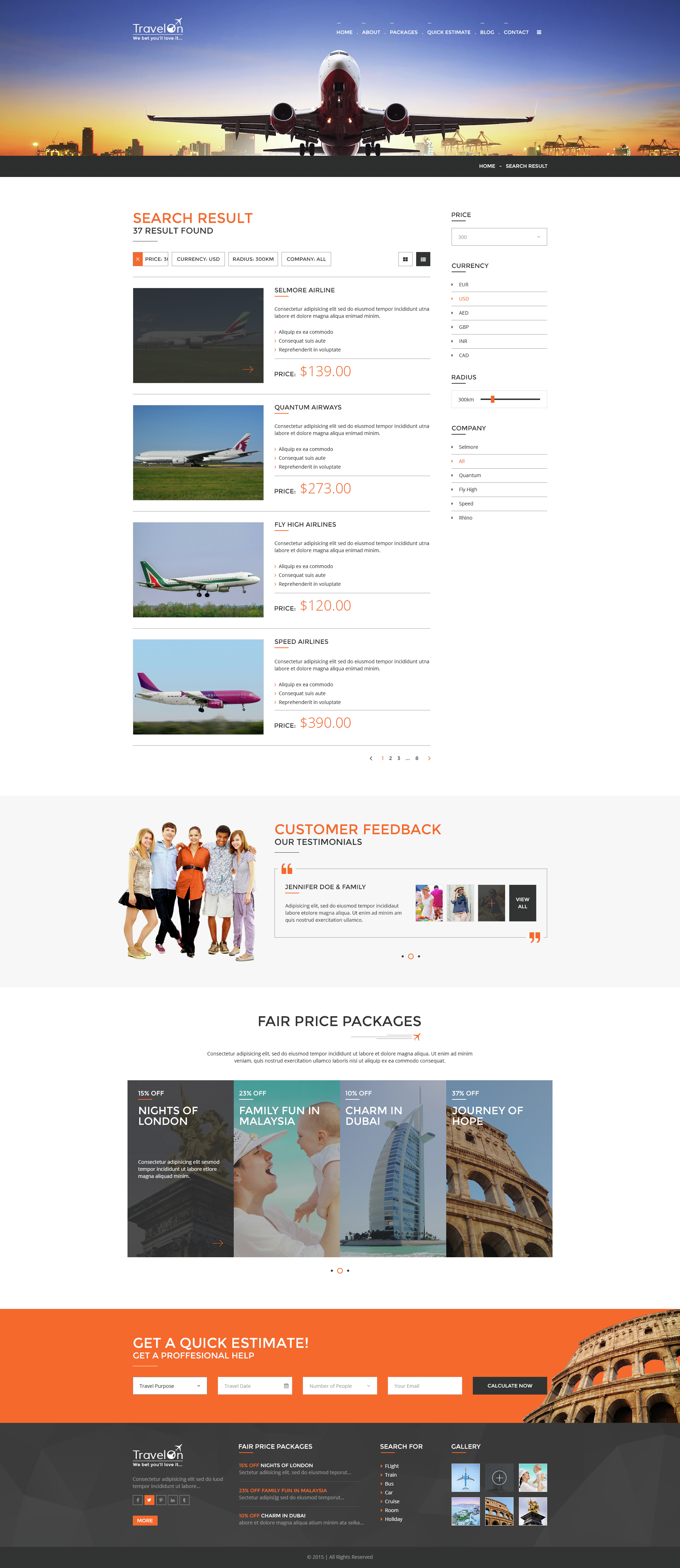The homepage of this website appears to be designed for booking plane tickets, although it has been condensed to a smaller screen size, making most of its content difficult to read and somewhat blurry. At the top, there is a large banner displaying a prominent image of an aircraft situated at an airport during dawn, with a beautiful gradient of orange, yellow, and blue hues in the sky. Navigation buttons are present at the top, though they are too small to decipher.

Below the banner, the section labeled "Search Results" lists several entries, though the details are similarly blurred. Four pictures of different aircraft are displayed, each with accompanying text that is also unreadable. The prices, displayed in red next to each picture, are mostly illegible due to the blurriness.

Additionally, there is a distinct box featuring a group of people standing together, labeled "Customer Feedback," which seems to be an advertisement. Another ad appears at the bottom of the page, showing images of the Roman Colosseum, another landmark, and a mother holding a child.